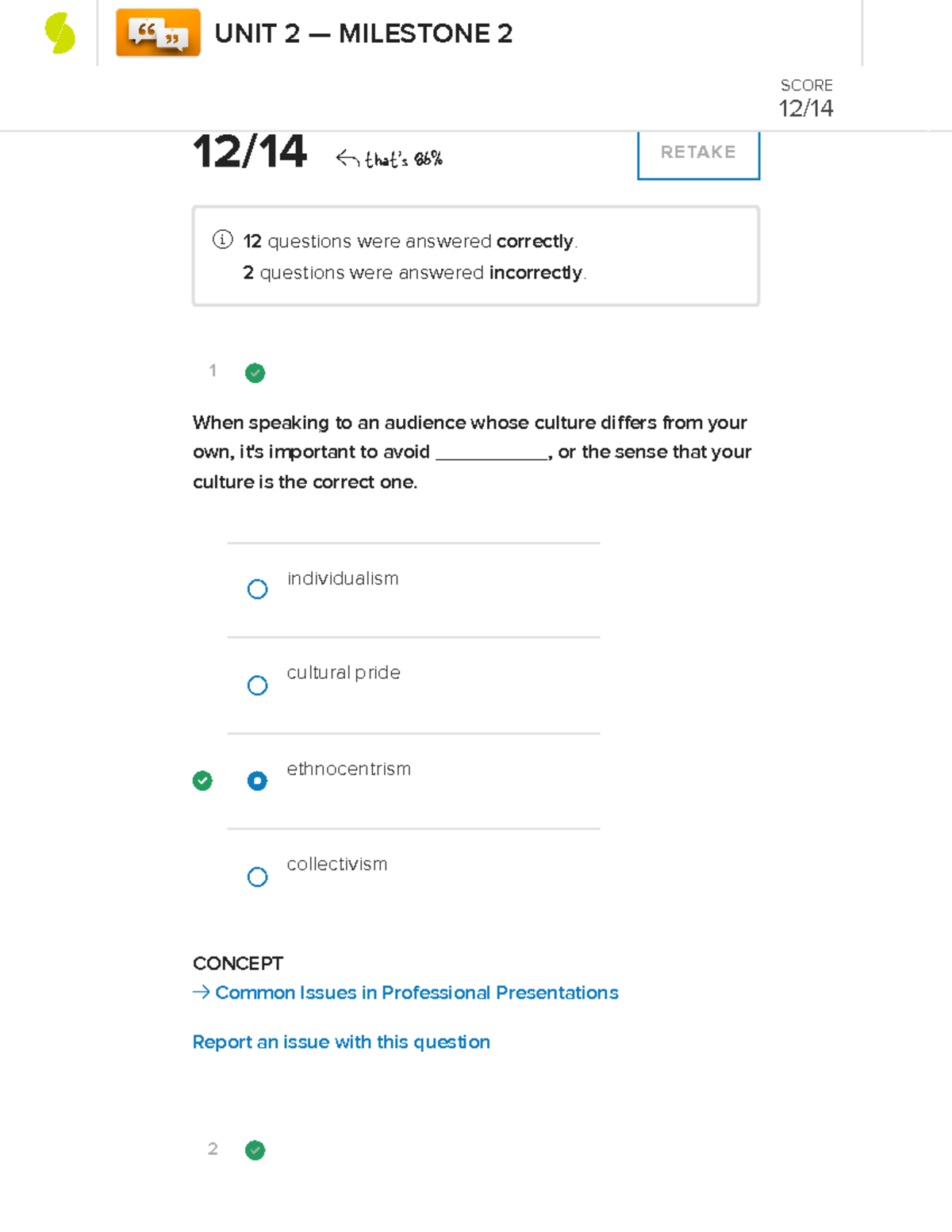The image appears to be a screenshot of a test or assignment evaluation sheet for Unit 2, Milestone 2. At the top right corner, it prominently displays a score of 12 out of 14, along with a calculated percentage of 86%, indicated by an arrow. On the right-hand side, there is a "Retake" button. 

A detailed performance summary reveals that 12 questions were answered correctly, while 2 were incorrect. 

The visible question reads: "When speaking to an audience whose culture differs from your own, it's important to avoid blank or the sense that your culture is the correct one." The answer choices provided are:
- Individualism
- Cultural Pride
- Ethnocentrism
- Collectivism

The correctly selected answer, "Ethnocentrism," is marked with a blue circle and additionally validated by a green circle with a checkmark. 

Below the question, it mentions the broader concept addressed: "common issues in professional presentations." There's also an option to report an issue with the question, suggesting user feedback functionality.